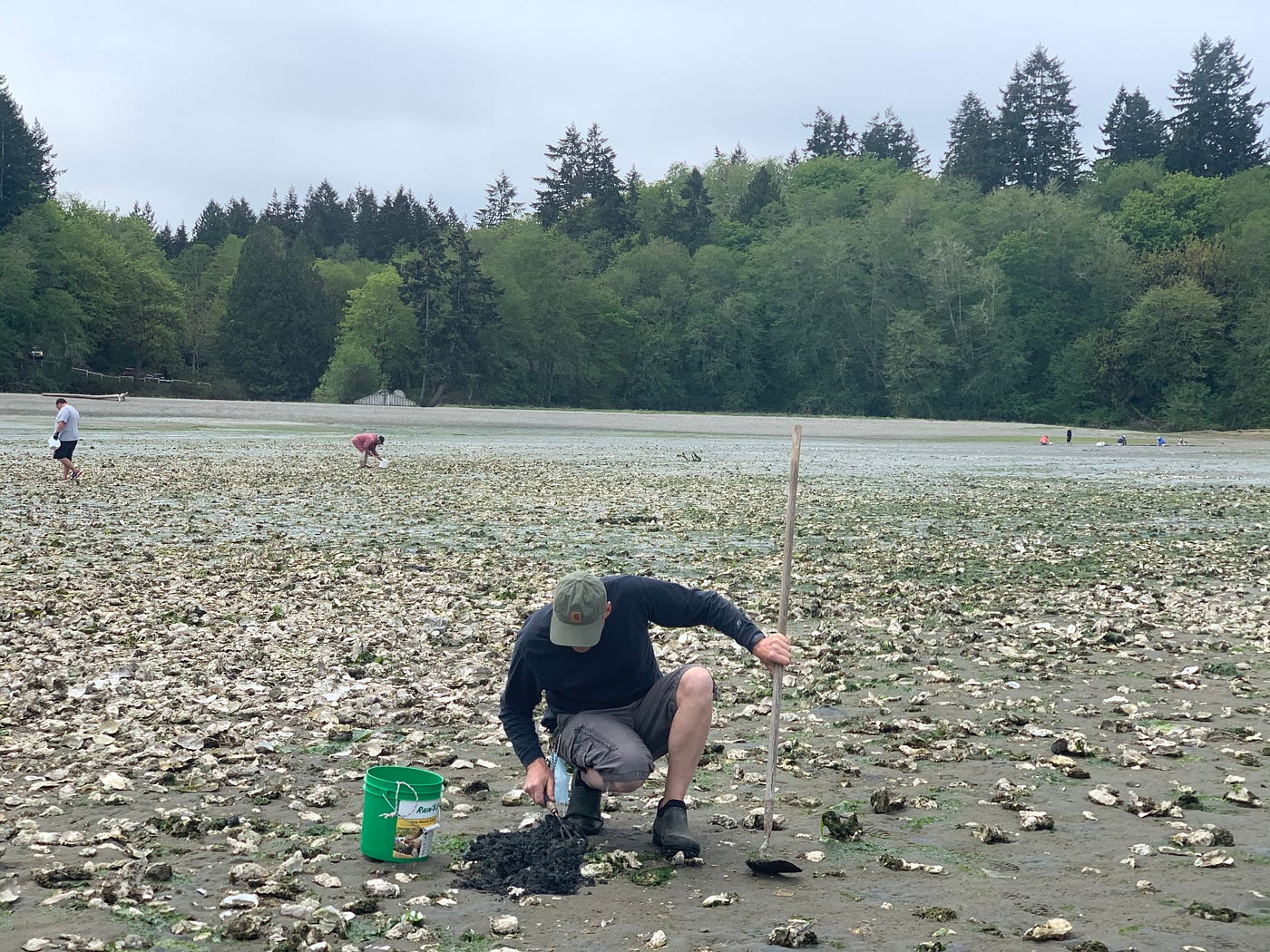In this horizontally-oriented photograph taken outdoors during the day, we observe a diverse scene featuring several individuals engaged in an activity, possibly collecting or cleaning up debris in an open field bordered by a forest. The sky above is light blue with gentle white clouds, and the horizon is marked by a dense tree line composed of trees in varying shades of green, both deciduous and evergreen.

Dominating the foreground is a Caucasian man kneeling on his heels. He is wearing a sage green Carhartt baseball cap, a long-sleeved blue top, gray cargo shorts, and black Crocs. With a focused demeanor, he uses a handheld three-pronged garden rake in his right hand to sift through dark, muddy material, which could be soil or organic waste. In his left hand, he holds a taller hoe, while a green bucket is positioned to his left.

Scattered across the muddy and leaf-strewn field, short green grass and possible puddles can be seen. Other individuals populate the midground and background. To the left, a man in a gray t-shirt and black shorts walks, carrying a white bag and looking down as if searching for something. Near the center-left, a figure in a reddish-pink coat bends over, seemingly inspecting or collecting something. To the far right, a group of about six people can be spotted, some sitting and others standing, dressed in various colors including pink, black, white, gray, and blue. These individuals are interacting with the field and its debris, contributing to the sense of a collective task being underway.